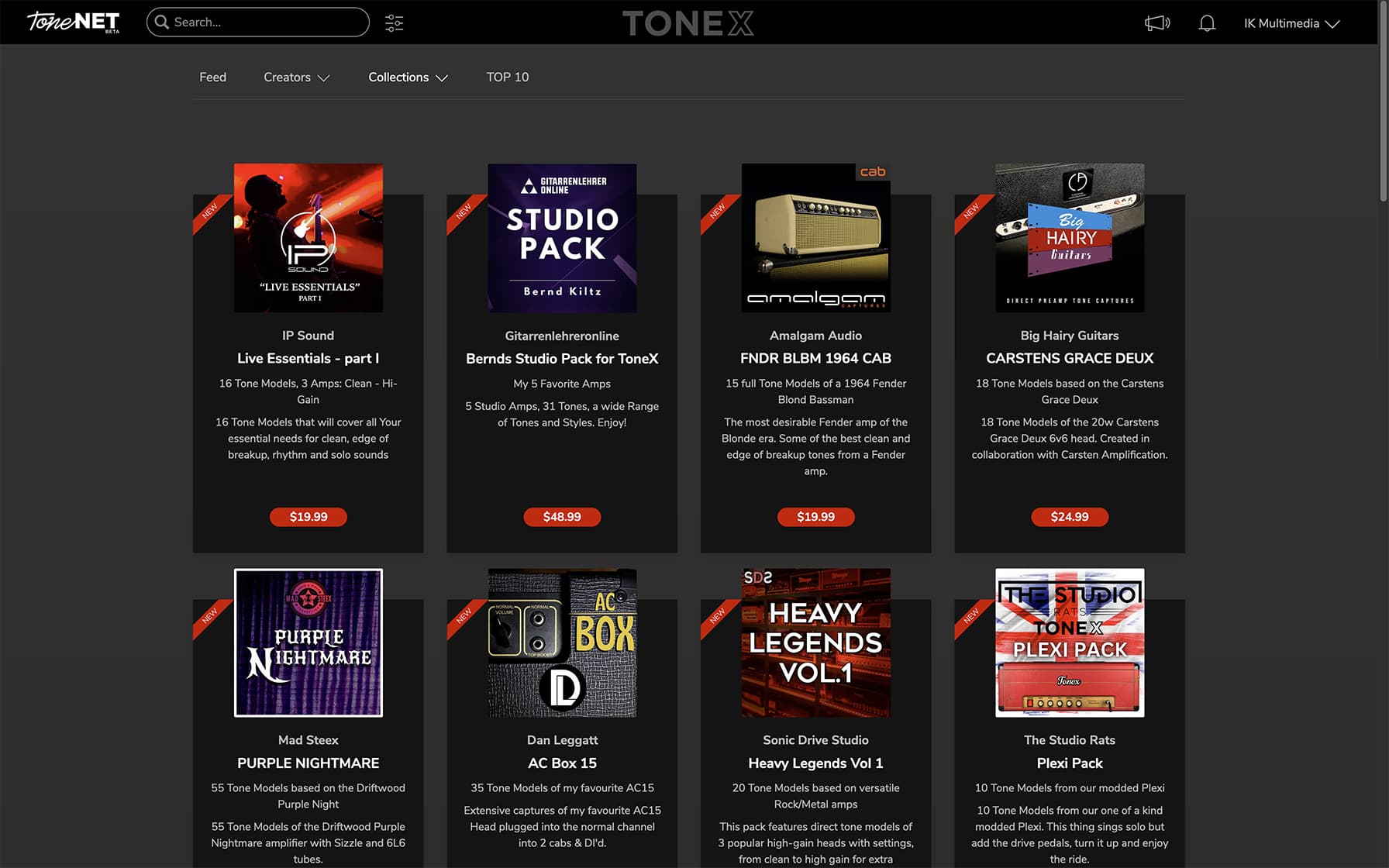A screenshot is displayed from the website Tone.net, showcasing various packages, although the text on the packages is illegible due to the small size. The overall theme is monochromatic, dominated by black and grayscale tones. At the center of the screenshot, the Tone X logo is prominently featured. The website includes a search bar at the top, with a sleek, modern design that features black tiles as the background.